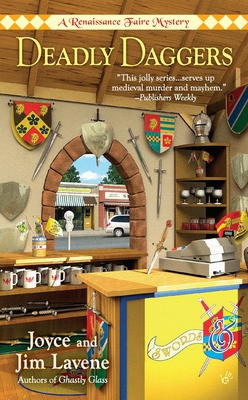The cover of "Deadly Daggers: A Renaissance Faire Mystery" by Joyce and Jim Lavene, authors of "Ghastly Glass," features an intricately detailed illustration of a Renaissance Faire booth. At the top, the tagline "A Renaissance Faire Mystery" sits above the title "Deadly Daggers" in yellow text, with a quote from Publishers Weekly describing the series as serving up "medieval murder and mayhem." The booth is filled with Renaissance-themed merchandise, including mugs, goblets, and a helmet on a corner shelf. The walls are decorated with an array of swords and shields in various colors, including red, green, yellow, and silver. A modern cash register sits on a counter adorned with coats of arms. Through an open archway, the contrast of modern life is visible with regular buildings, shops, and a silver car seen in the distance.